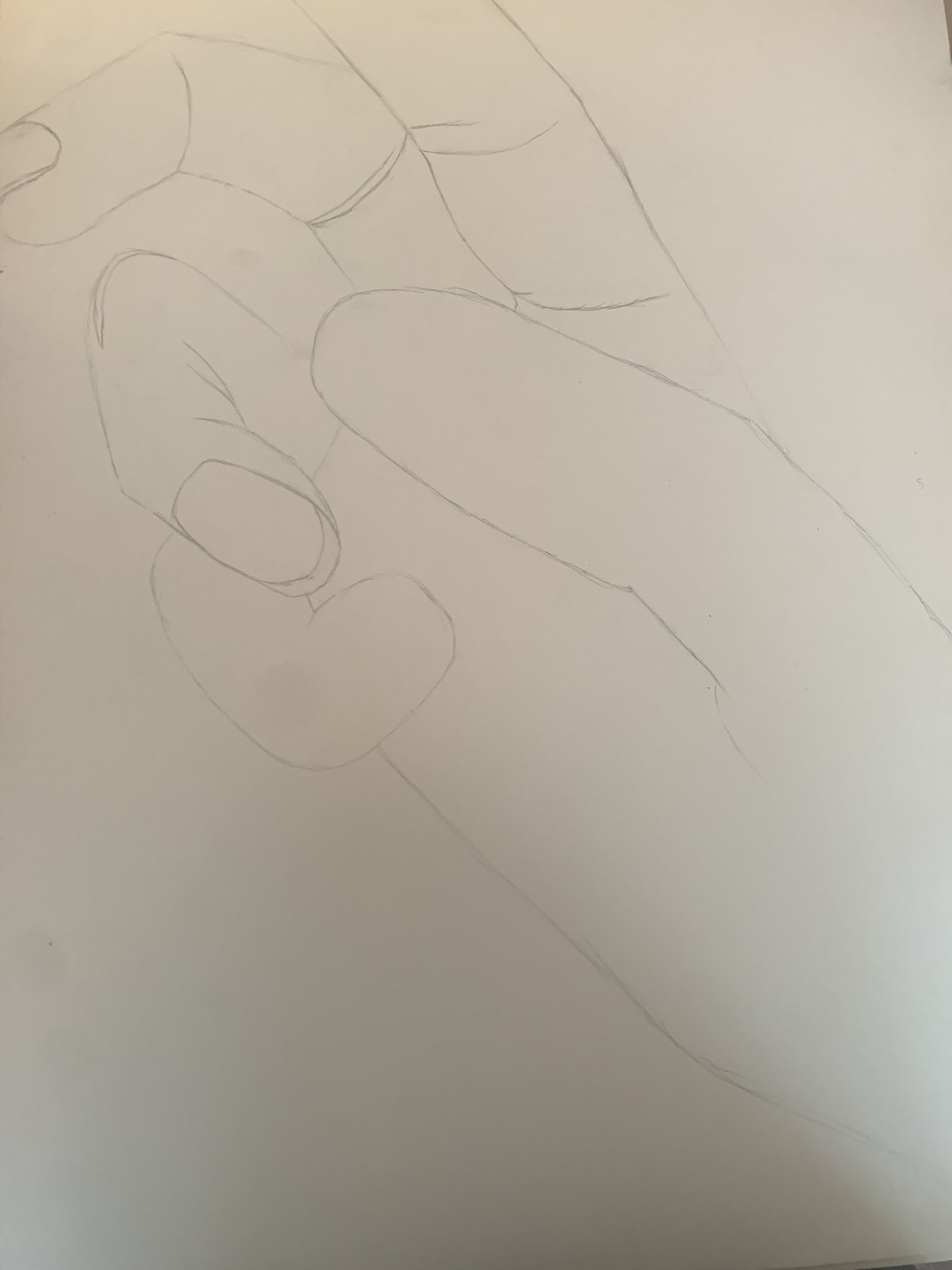The image depicts a detailed pencil sketch on a white sheet of paper, featuring a highly realistic drawing of a hand extending from the bottom right corner of the page. The hand is shown from the bottom of the palm up to the tips of the fingers, with a slight grey gradient shading at the bottom. The index finger points straight up, while the thumb is bent underneath the hand, and the pinky is tucked underneath the ring finger in an L-shape. The middle and ring fingers have visible fingernails, whereas the thumb and pinky lack any nail detail. The hand appears to be almost seamlessly connected to the wrist without any distinct break lines. The hand and fingers, though meticulously outlined, remain unshaded and filled in pure white, contrasting sharply with the grey tones of the drawing. Aside from the hand, there are no other prominent details or text visible in the image, except for a subtle and ambiguous hint of a table corner at the top right.